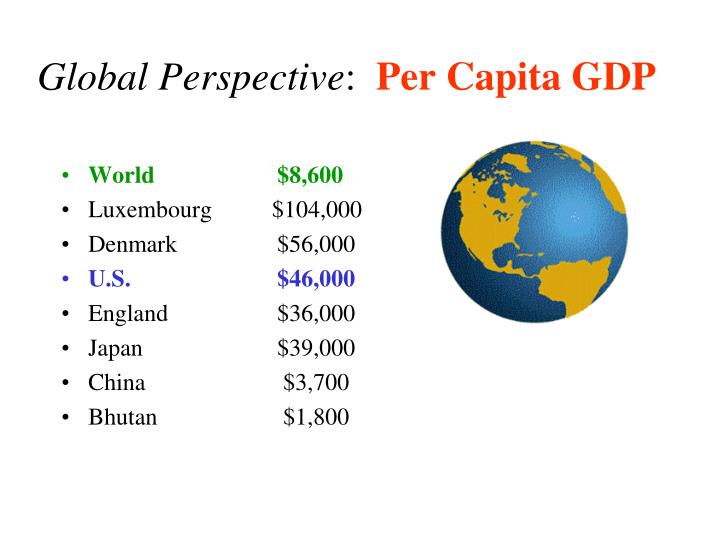The image appears to be a detailed presentation slide with a white background, titled "Global Perspective: Per Capita GDP." The title is written in black text for "Global Perspective" and red text for "Per Capita GDP," using different fonts. Below the title, there is a bulleted list of countries with their corresponding per capita GDP figures. The list starts with "World" in green text, indicating a per capita GDP of $8,600. Following are:

- Luxembourg: $104,000
- Denmark: $56,000
- U.S.: $46,000 (in blue text)
- England: $36,000
- Japan: $39,000
- China: $3,700
- Bhutan: $1,800

All figures are in black text except for "World" and "U.S." To the right of the list, there is a clip art image of the Earth, depicting the globe with yellow land masses and blue oceans.